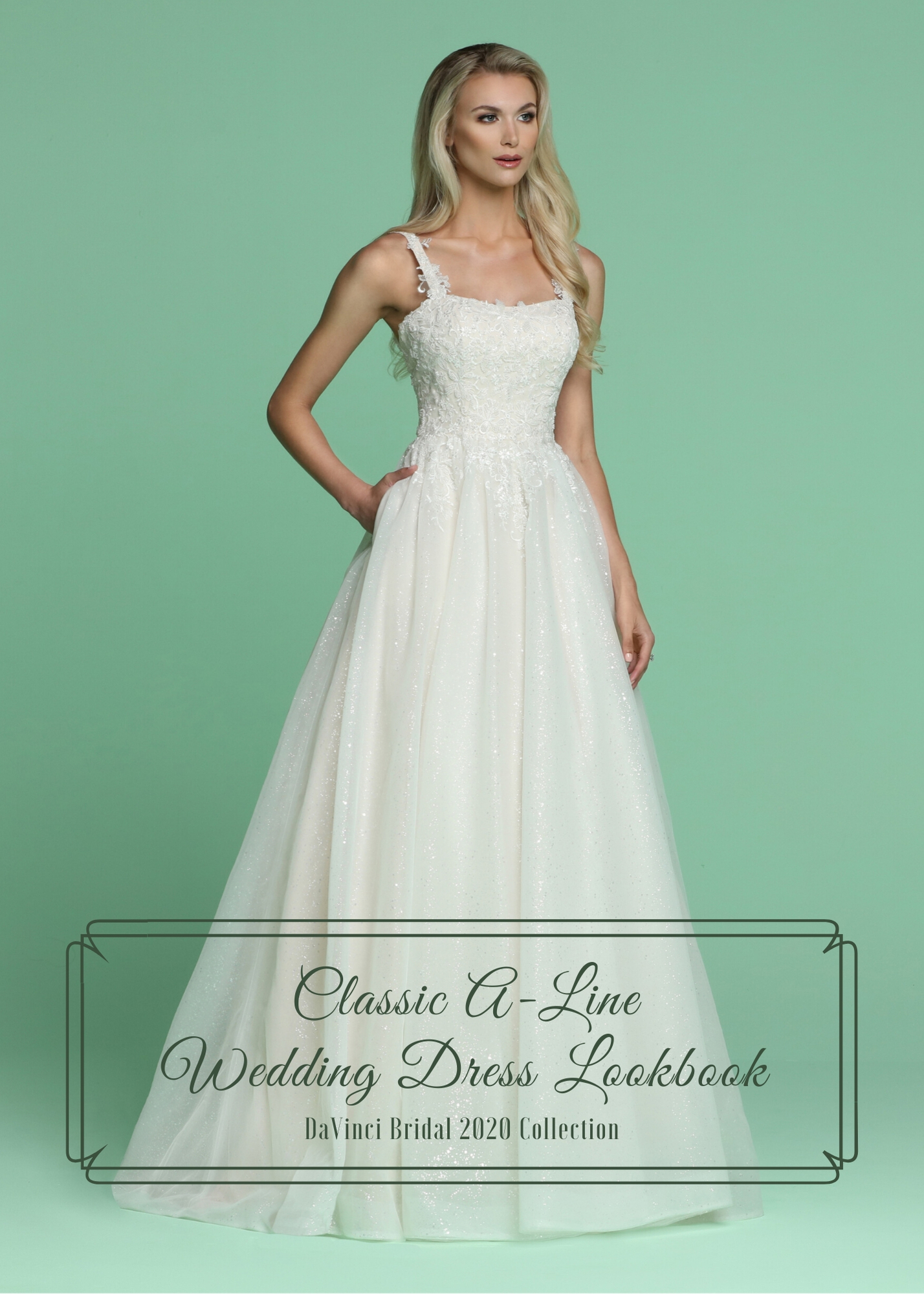The image is an advertisement showcasing a woman in a classic A-line wedding dress from the Da Vinci Bridal 2020 Collection. The dress is sparkling white and has straps, revealing her shoulders, neck, and the top of her chest and arms. The woman has long, wavy blonde hair and is wearing lipstick, with her mouth slightly open and one hand on her hip. She is looking slightly off to the right, standing in front of a dark pastel green backdrop with a lighter pastel green floor. Over the image, a black rectangle with a clover shape contains the text in cursive black font: "Classic A-Line Wedding Dress Lookbook, Da Vinci Bridal 2020 Collection."